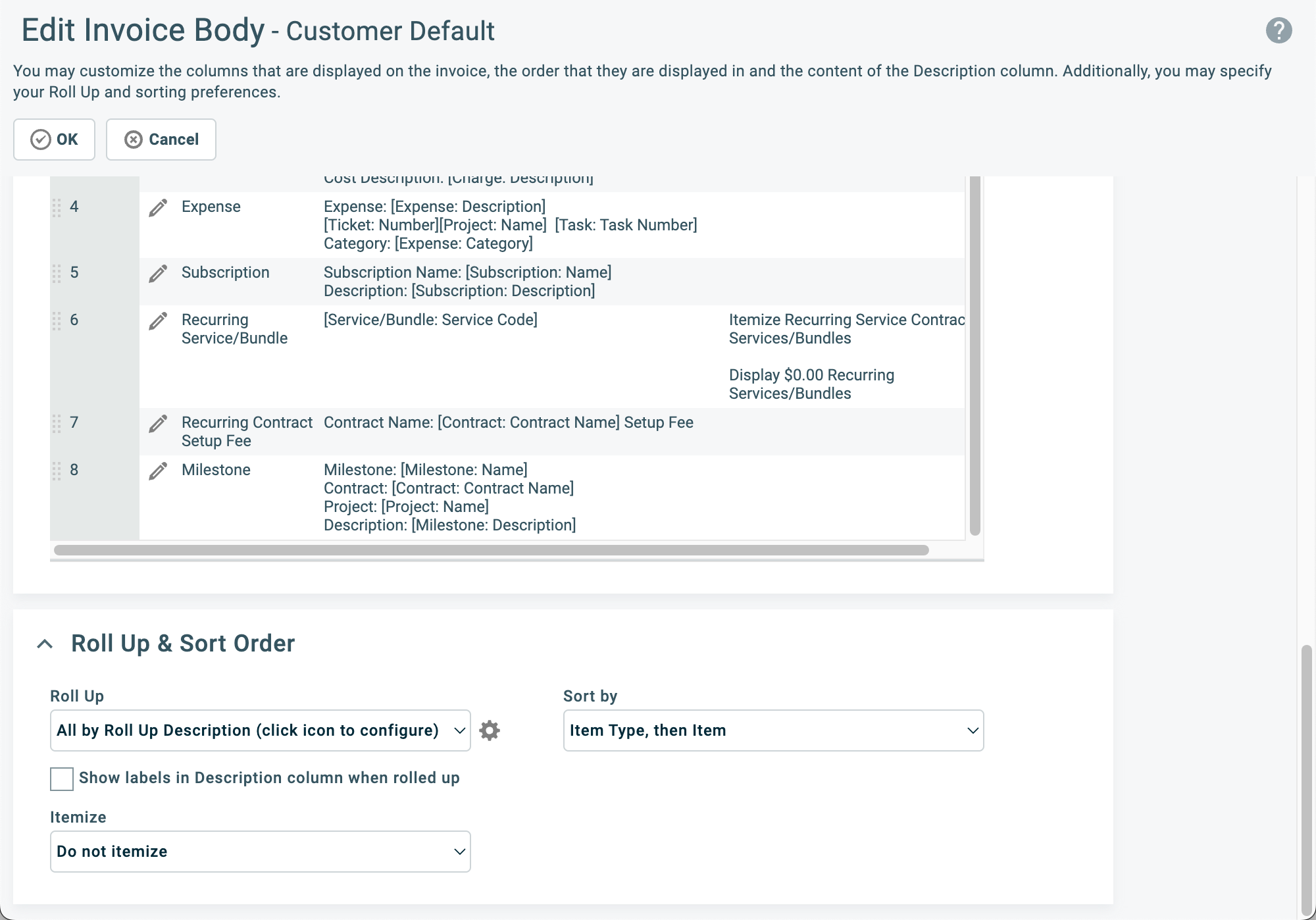This screenshot displays an interface for editing an invoice body, set against a light gray background. In the upper left corner, bold black text reads "Edit Invoice Body, Customer Default." Below this, in smaller black text, there's a description: "You may customize the columns that are displayed on the invoice, the order that they are displayed in, and the content of the description column. Additionally, you may specify your roll-up and sorting preferences."

Two white buttons, labeled "Okay" and "Cancel" in black text, are situated below this text. At the bottom, a section labeled "Roll-Up and Sort Order" is presented in black text against a white background. This section includes a dropdown menu labeled "Roll-Up" with the prompt "Click icon to configure" and an option to "Show labels in description column when rolled up." Beneath, there's another dropdown menu with the option "Do Not Itemize."

In the upper right of this white section, there’s an area for sorting preferences. It has a label "Sort By" and features a dropdown menu that currently displays "Item Type," followed by another dropdown showing "Item."